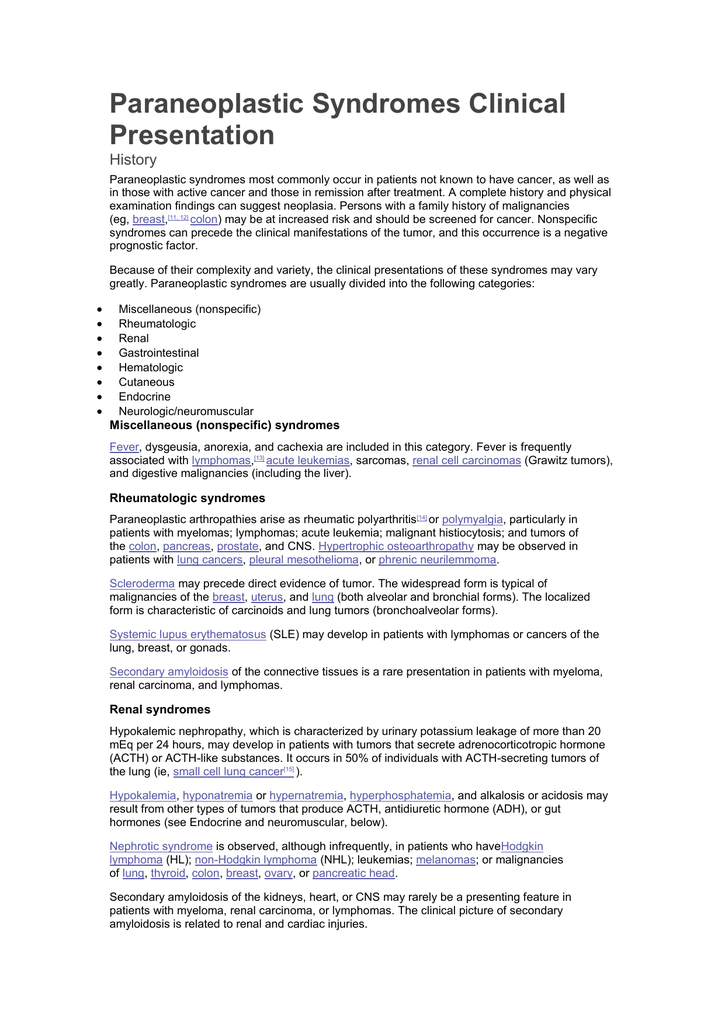In the image, we see an article about "Paraneoplastic Syndromes: Clinical Presentation," with the title prominently displayed in bold, dark font. Below the title, the section heading "History" is presented in a smaller font, followed by the main body text, which discusses the clinical features and history of paraneoplastic syndromes. The article begins with an introductory paragraph that explains the concept of paraneoplastic syndromes. Following this, the text transitions into a detailed exploration of different types of these syndromes.

Highlighted portions of the text are emphasized in blue with underlines, indicating that they are hyperlinks that provide additional information or redirect to external sources for further reading. The article contains bullet points that list the symptoms associated with paraneoplastic syndromes, making it easier to read and comprehend. Notably, blue-highlighted areas within the bullet points also link to further explanations or resources for those terms.

Towards the end, the article concludes with a discussion that may involve potential injuries linked to paraneoplastic syndromes, with the word "injuries" appearing as the final word. The layout and presentation are designed to provide a thorough and accessible overview of the condition for readers, complete with interactive elements for deeper exploration.